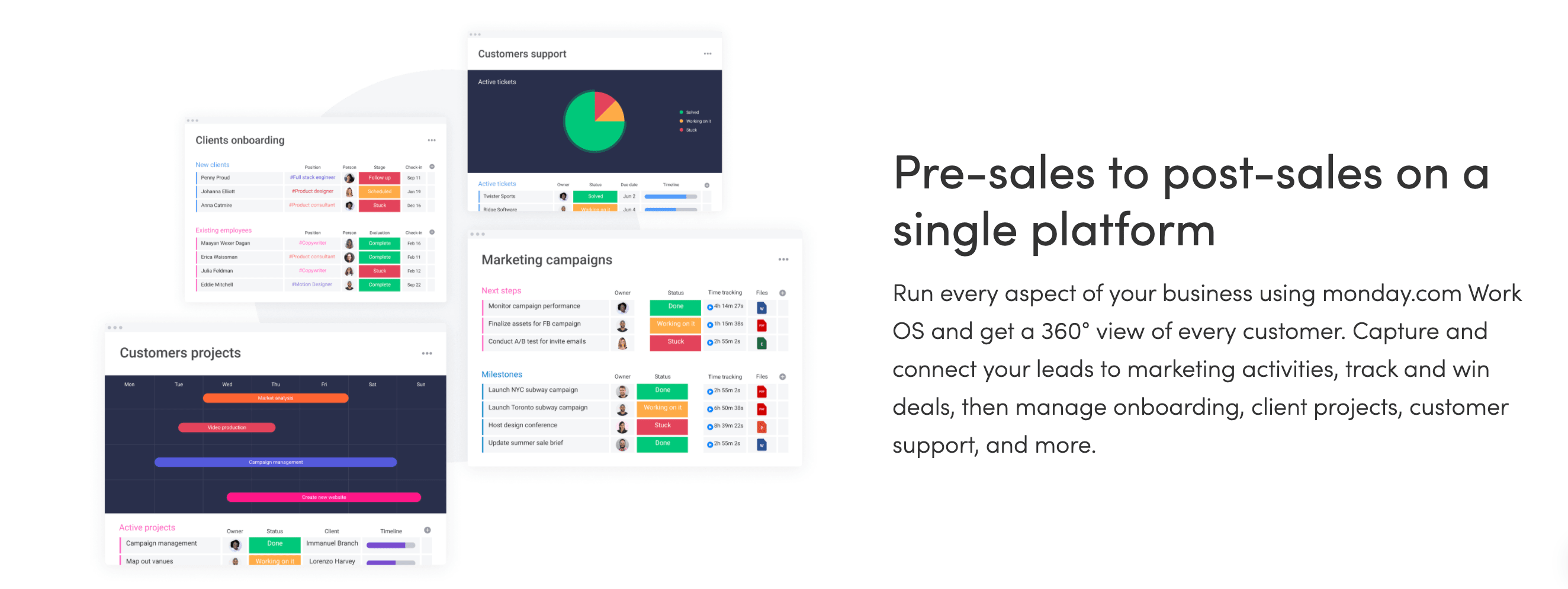This is a sequence of rectangular images set against a white background, with a large, light blue circle partially visible behind each image. At the top of the series is an image featuring a pie chart. This image consists of a white banner at the top, followed by a mostly navy blue background. In the center is a pie chart colored in green, red, and yellow with a small, difficult-to-read key on the side. The majority of the pie chart is green, while the remaining sections are evenly divided between red and yellow. Below the pie chart, there is more information, which is also too small to decipher. 

Beneath this image, there is another rectangular image. This one is labeled "Marketing Campaigns" in black text at the top. It contains color-coded information, but again, the text is too small to read clearly.

The final image in this series has the heading "Customers Projects" in black text on a white background. The rest of the image has a navy blue background and features several colored bars of varying lengths. The bars are orange, red, blue, and pink, each with accompanying text that is too small to be legible.